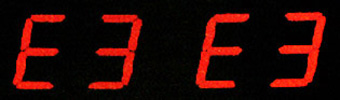The image displays a long, thin strip typical of a gauge, approximately four times as wide as it is tall, set against a completely black background. Centered within this strip are four bright red characters. The first character is a red uppercase "E" created by a horizontal line at the top connected to a vertical line on the left, continuing down into another horizontal line extending to the right, and finishing with a second vertical line leading to a final horizontal line to the right. Following this is a red numeral "3," formed by a sequence of horizontal and vertical lines: a horizontal line on top connected at the right by a vertical line descending into another horizontal line that extends left, and a final vertical line leading down to a bottom horizontal line ending to the left. This pattern—an "E" followed by a "3"—repeats itself, resulting in "E3 E3," all rendered in red against the stark black background.